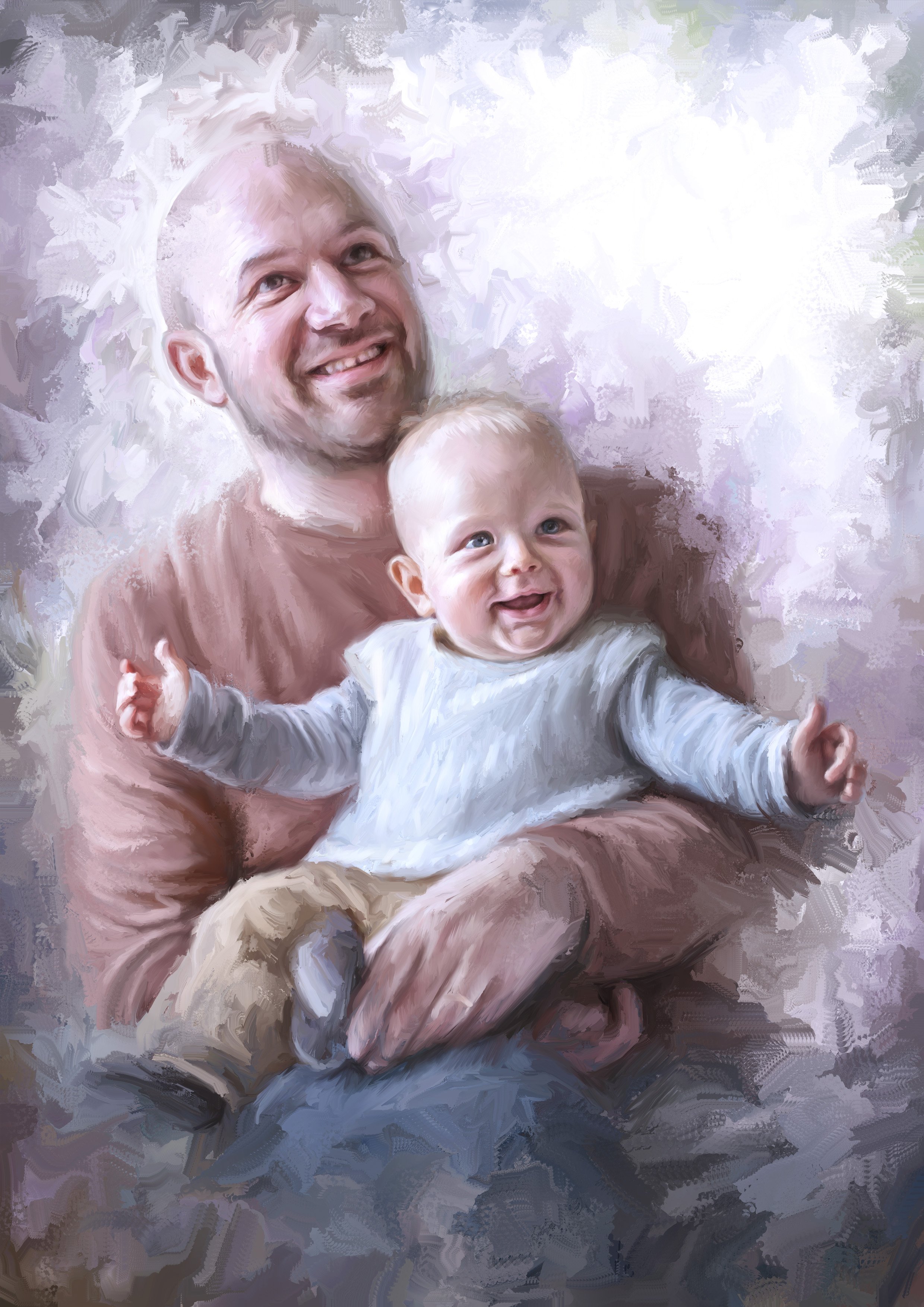In the image, a painting captures a joyful moment between a man and his baby son. The man, bald and smiling, gazes up and to the right while holding his son in his lap. His taupe or light brown/orange sweater contrasts with the smudgy gray and blue brushstrokes that form the background of this impressionist-style portrait. The baby, with blonde hair and blue eyes, looks slightly off-center and wears a light blue or gray sweater paired with beige or brown pants. Both figures appear happy, sharing a warm and affectionate bond. The scene is brought to life with large, dynamic paint strokes, leaving an impressionistic yet detailed depiction that raises questions about whether it was manually painted or digitally created. The baby sits comfortably on the man's lap, adding to the intimate and endearing nature of this family portrait.